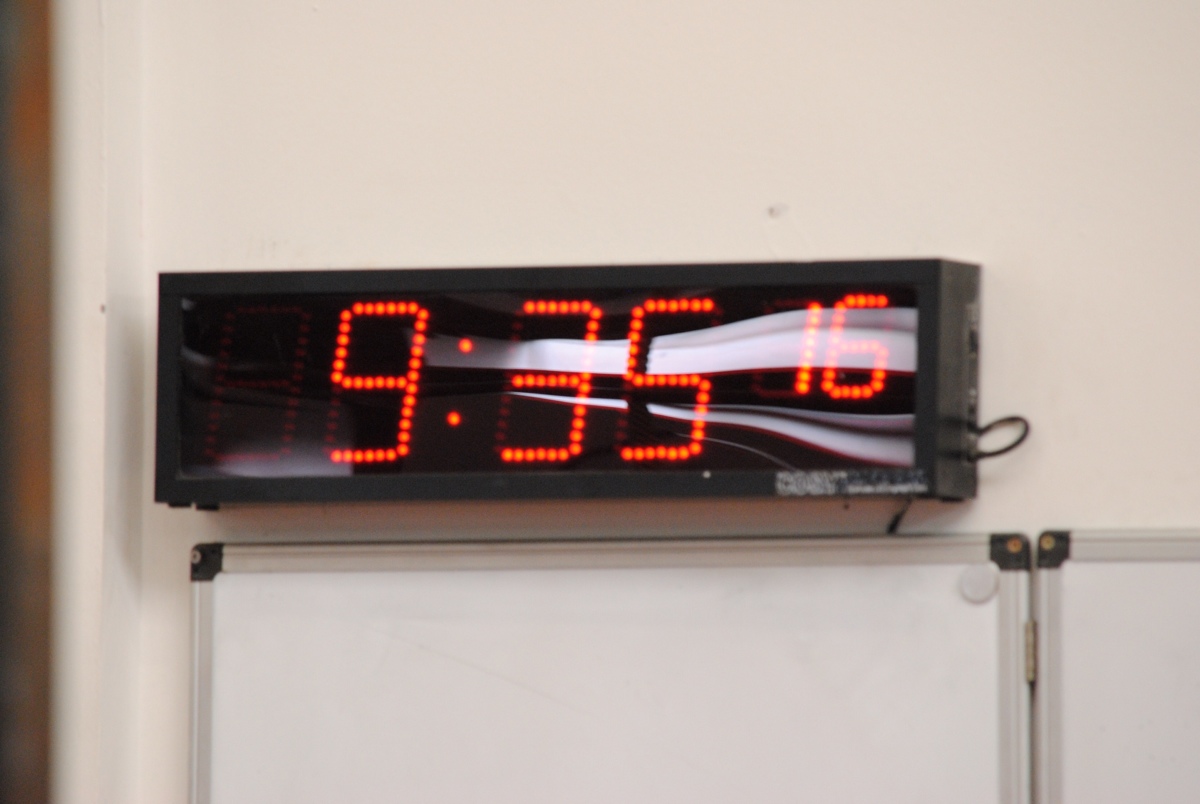This horizontally-aligned, portrait-oriented photograph captures the upper section of a doorway that features a rectangular LCD screen. The screen, set against a black backdrop, prominently displays red numbers "935" in large font and a smaller "16" beneath it. Due to significant glare, the details on the screen are partially obscured. Surrounding the screen, the background wall is painted an eggshell white, while the left side of the image reveals a section of dark wooden trim.